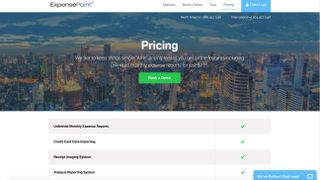This is a horizontal rectangular image, somewhat small and challenging to read. At the top of the image, there is a logo positioned slightly to the right of the left edge, approximately halfway between the left edge and the center. The logo seems to start with the letters EXP, although it's difficult to discern clearly.

To the right of the logo, there are five menu items listed in a black font, with the final one featuring a turquoise background and white text. Below this menu section is an image that appears somewhat dark. The image depicts a densely packed cityscape filled with numerous tall buildings and illuminated lights, suggesting a bustling urban environment.

In the middle of the image, the word "Pricing" is prominently displayed in bold white font. Below this title are two lines of additional white text, followed by a green horizontal rectangular section with unreadable white font within it.

Continuing downward, four lines of text alternate between light gray and crisp white, all presented in bold black font. Each line has a green checkmark on its right side. The final line includes an additional turquoise horizontal rectangle extending into the white area, containing white text that is also difficult to read.